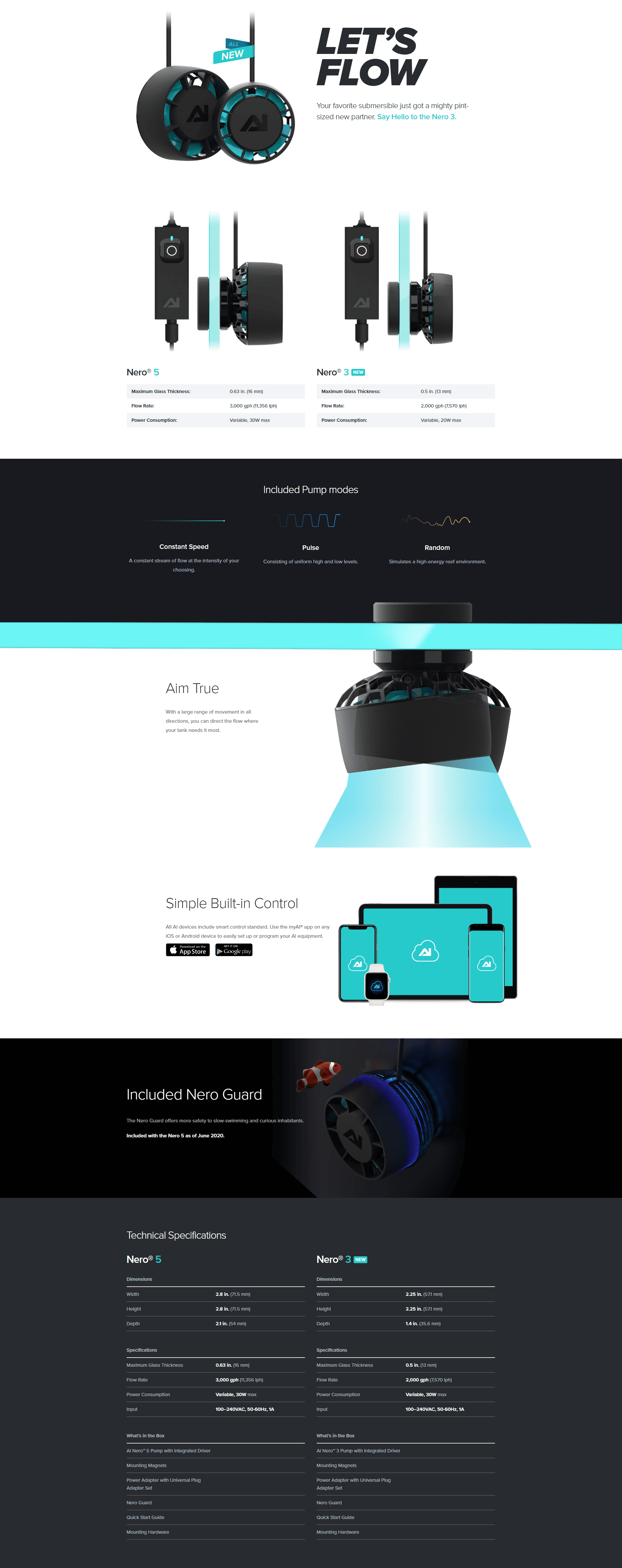In this image, we see a detailed advertisement prominently featuring a sleek electronic device. The webpage appears zoomed out, providing a comprehensive view of the layout. At the very top of the image, the bold slogan "Let's Flow" is displayed, setting a dynamic tone. The electronic device showcased is primarily black, accented with a subtle light blue tint and emanating a radiant light blue glow.

Beneath the tagline, a black section is segmented into three categories, each clearly labeled in white text. A thin, light blue line runs horizontally across this section, creating a visual divide. Below this, the device itself is positioned, capturing attention with its striking black design illuminated by blue light.

The background of the ad is predominantly white, offering a clean and modern aesthetic. Scattered below the main device are multiple screens, including two tablets and two cell phones, arranged artistically to emphasize the product's versatility.

Further down, another section with a solid black background features finely printed white text, likely detailing additional product specifications or promotional information. At the very bottom, the image transitions to a gray background filled with numerous columns of extremely small white text. These columns, arranged three per section, provide extensive information about the product, concluding the detailed advertisement from top to bottom.